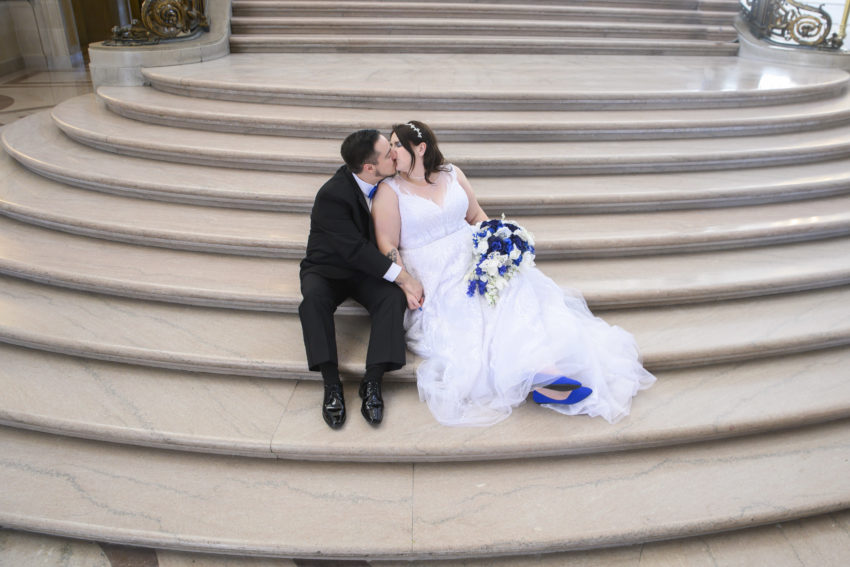This photo captures a tender moment of a newlywed couple seated on a large, ornate marble staircase. The groom, dressed in a black tuxedo with a white undershirt and blue tie, is kissing his bride, who is wearing a flowing white wedding dress. She holds a stunning bouquet of white and blue flowers in her left hand and has blue high heels peeking out from beneath her gown. Her brown hair is adorned with a sparkly headband. The groom has short, dark hair, sideburns, and a thin beard, and he is wearing black dress shoes and black socks. The staircase, made of tan-colored marble, features intricate railings and pillars, adding to the elegance of the setting. This beautifully ornate backdrop enhances the intimacy and warmth of their shared kiss.